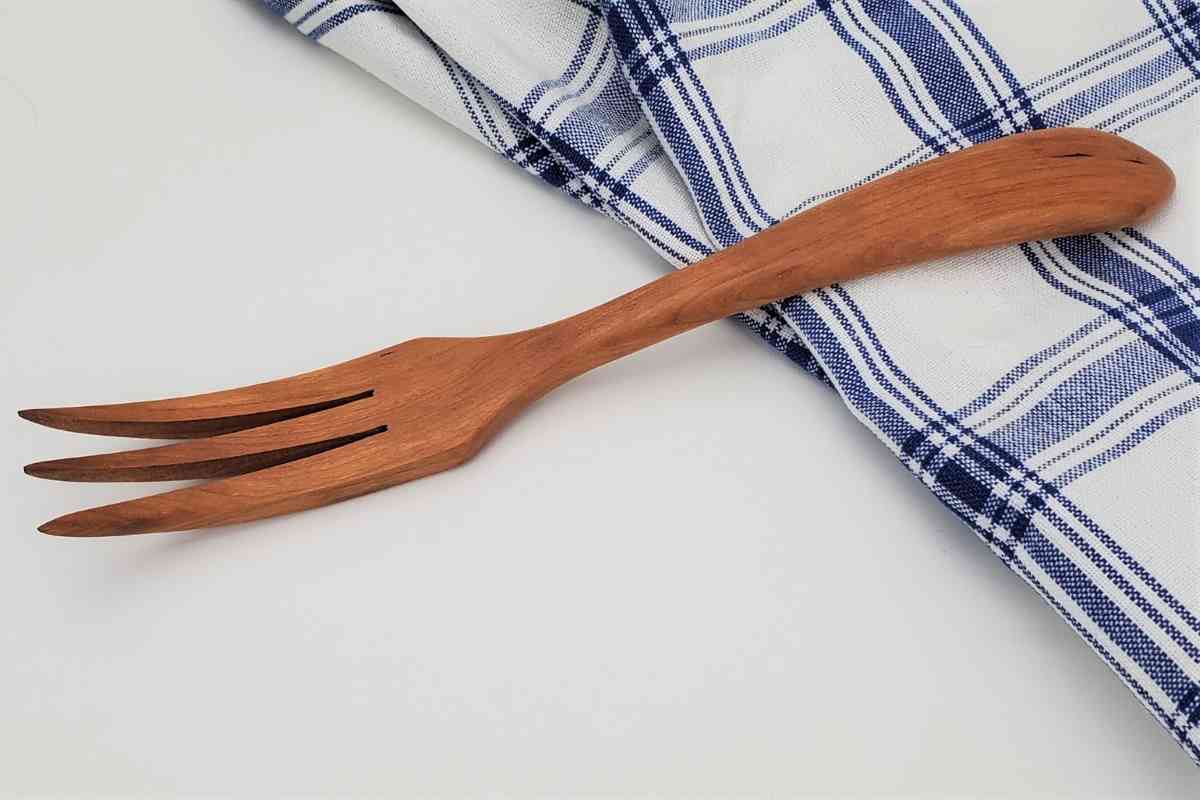The photograph displays a handcrafted wooden fork, predominantly brownish-red in color, positioned diagonally from the upper left-hand corner to the middle right-hand side of the image. The top portion of the fork rests on a blue and white checked tablecloth, notably described with alternating dark blue and thin stripes, forming a plaid pattern. The bottom tip of the fork, featuring three pointed tines, rests on or near a plain white surface, likely a table or counter. The fork itself, which has a darker hue at the tips of the tines, appears to be crafted from a wood such as teak or cedar. The handle begins on the fabric and extends onto the table, creating a sense of depth as the tines angle slightly upwards. This rustic utensil is reminiscent of a salad or mixing fork, commonly used in various culinary settings.